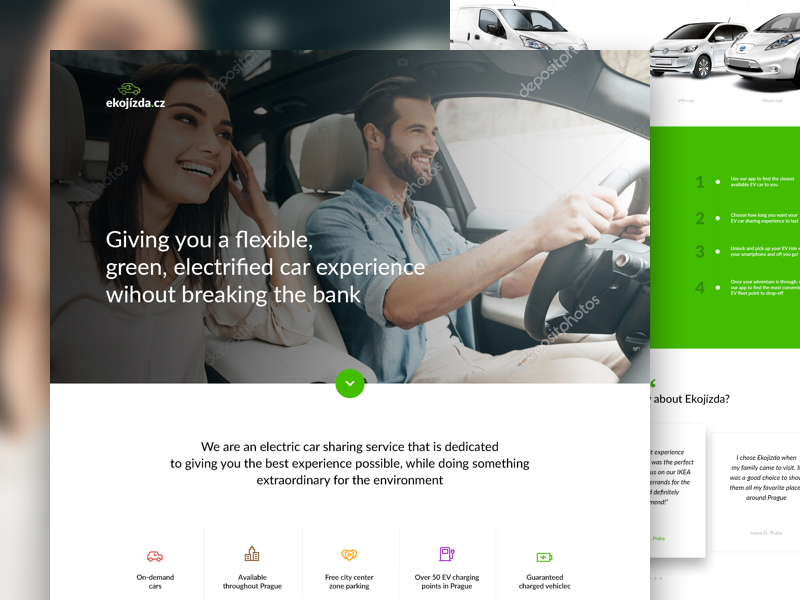This website screenshot showcases the homepage of E-K-O-J-I-Z-D-A (ekojižda.cz), an electric car-sharing service based in Prague. At the very top, the website's URL is prominently displayed. 

The main visual element is a photograph featuring two young individuals in a car. The woman seated in the passenger seat has long dark hair, is looking forward with a cheerful smile, and rests her left hand on the side of her head. The driver, a young man with short dark hair complemented by a mustache and beard, is also smiling as he looks straight ahead. He wears a blue denim shirt with the sleeves rolled up to his elbows and has both hands on the steering wheel.

Accompanying the image, a promotional blurb highlights the service’s commitment: "Giving you a flexible, green, electrified car experience without breaking the bank." The text emphasizes that the electric car-sharing service aims to provide an exceptional user experience while contributing positively to the environment. 

Additional features of the service include on-demand cars available throughout Prague, free parking within the city center zone, over 50 electric vehicle (EV) charging points across Prague, and guaranteed charged vehicles.

On the top right of the screenshot, a partial photograph of several silver or white cars is visible, along with a segment of green text that provides a step-by-step guide:
1. Use the app to find the closest available EV car.
2. Choose the duration of your EV car-sharing experience.
3. Pick up your EV ride.
4. Once your adventure is through, use the app to locate the most convenient EV fleet point for drop-off.

However, some text appears too small and blurry to read clearly. The right side of the screenshot is partially obscured by the window on the left.